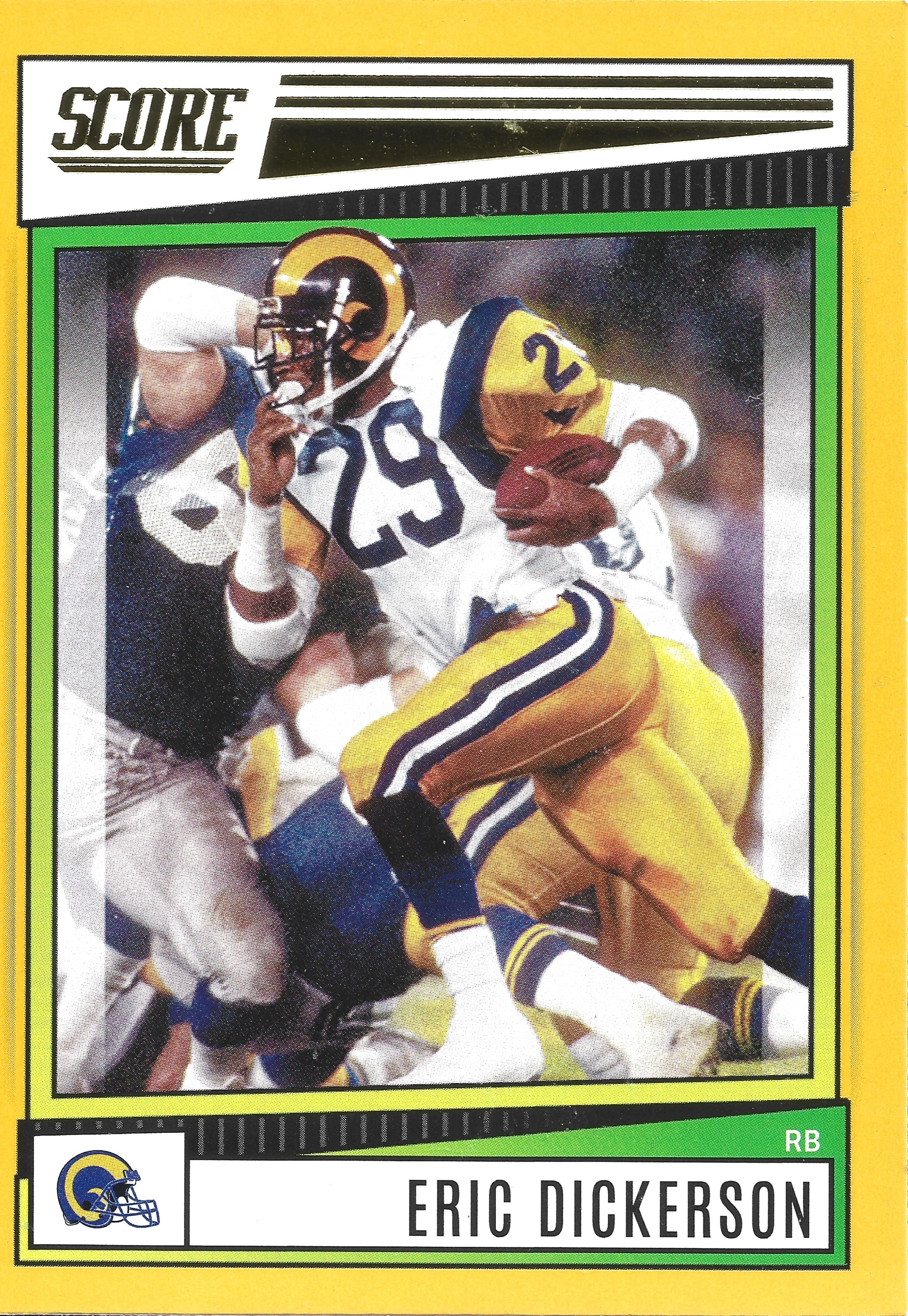This detailed football collector's card features a vibrant yellow border and a distinctive design. At the top of the card is a white and black rectangular banner, with the word "SCORE" prominently displayed in bold black capital letters in the upper left corner, underlined with two black lines, alongside three lines and a thick triangle on the right side. Below this, a green-outlined action shot showcases a football player, Eric Dickerson, in full stride running left to right. Dickerson wears a black and gold helmet, a white jersey with navy blue and gold accents, and gold pants with a blue and white stripe, donning the number 29 in blue. He's holding the football in his left hand while his right hand is raised near his helmet. Around him, several players, including one in a blue jersey and white pants with a visible number six, are engaged in the play, indicating a dynamic in-game moment with players clashing and others in the background. At the bottom left of the card is an image of a Ram's helmet, and to the right, within a white panel, "Eric Dickerson" is printed in black letters, with "RB" (for running back) situated above his name.